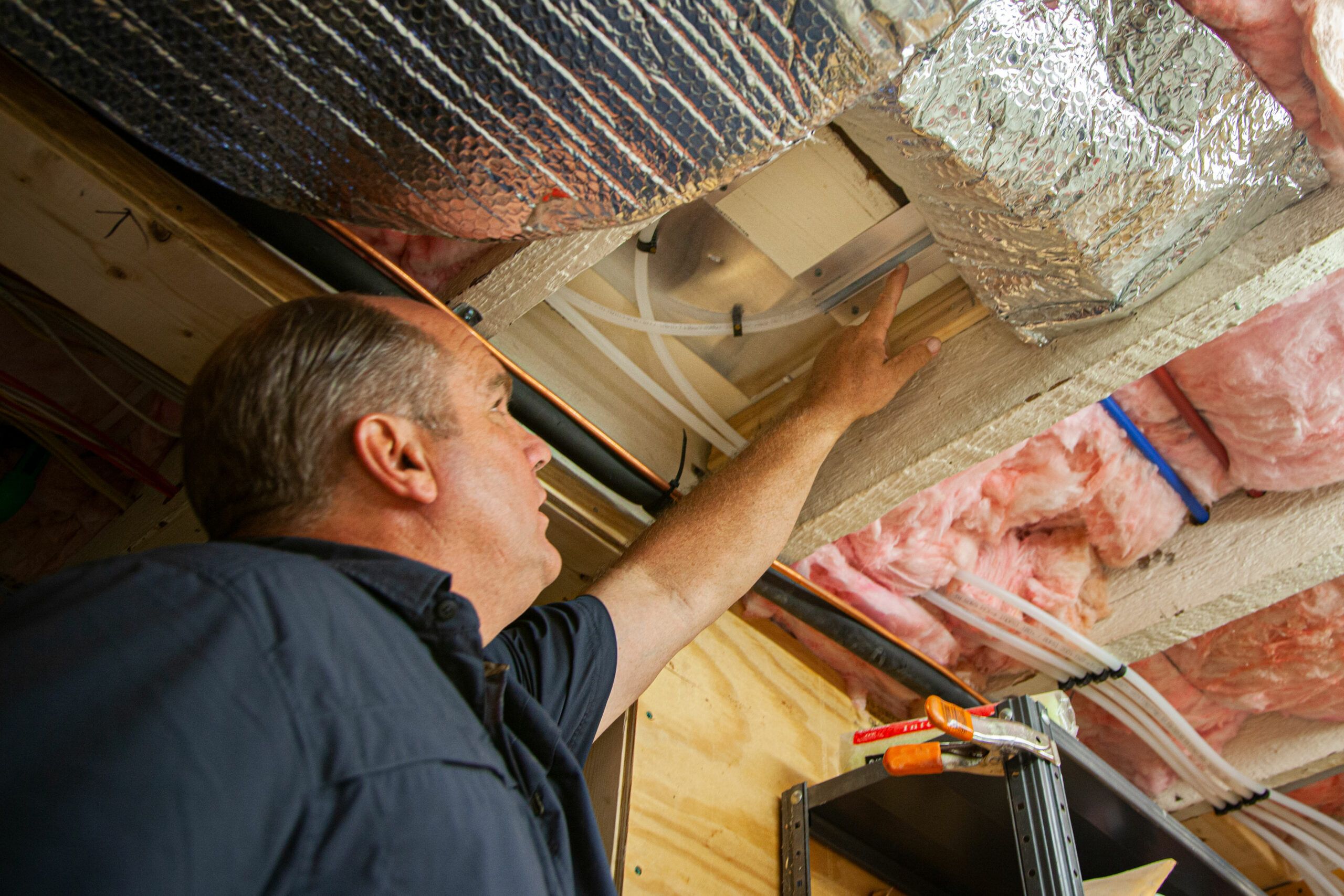The image depicts an older man with a very receding hairline, who is using his left hand to point at a specific water line among several that are exposed by folded-back insulation. The insulation is pink with a silver cover. This unfinished area reveals multiple water lines running in various directions. Notably, the man is specifically pointing to a blue water line, while the rest of the lines are translucent white, suggesting that the blue line might be of particular concern. These water lines, one of which curves off from a main setup, are all secured to the floor joists using plastic supports. Also visible in the image is an insulated line and an orange wire running through the same area.

In the background, a metal utility shelf can be seen with a clamp on top, indicating some temporary use or reference point for the man as he inspects the plumbing. His focused gaze and pointed gesture suggest there is a problem with the water lines that requires attention.